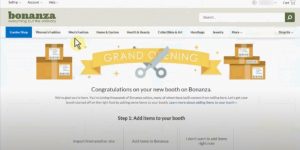This image depicts a screenshot of a website’s homepage, featuring several elements that are somewhat difficult to discern due to the small size of the image. In the upper left-hand corner, although not at the very top, the word "Bonanza" is clearly visible, printed in lowercase black font within a gray rectangular bar spanning the width of the page. To the right of this gray bar is a search feature, consisting of a white search box with the word "search" in gray font on its edge, followed by a white magnifying glass icon enclosed in a black box at the end of the bar.

Below this gray bar, a series of dropdown menus extends across the width of the website, although the text within these menus is too small to be legible. Further down, there are illustrations of a few stacks of boxes. Adding a touch of celebratory flair, a golden banner adorned with the words “Grand Opening” stretches partway across the page. This banner is complemented by a graphic of cartoon-like scissors poised to cut a symbolic grand opening ribbon.